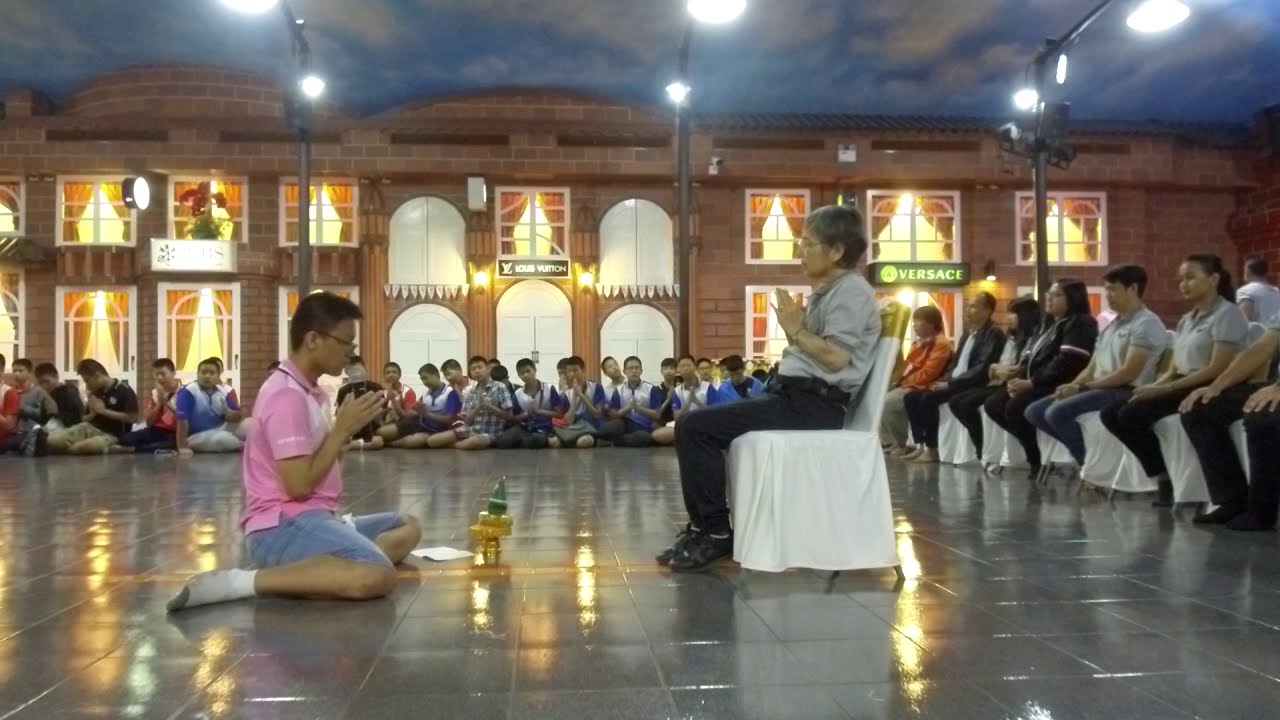The image is a photorealistic photograph taken inside a uniquely designed building. The far wall is painted to resemble a continuous brick facade of a city street, complete with stylized windows and doorways. Prominent signs adorn the pseudo-building, including a white sign on the left, a black Louis Vuitton sign in the middle, and a green Versace sign to the right. The ceiling is painted with a blue sky and white clouds, with ceiling lights suspended by long metal poles.

The floor is a shiny, reflective gray. In the foreground, near the left, a man in jeans and a pink shirt kneels with his hands clasped in a prayer position, directing his attention towards another person. This central figure, dressed in a gray shirt and black pants, sits on a white-covered chair. Both appear to be part of a ceremonial or instructional gathering.

Surrounding them is a large group of people, forming a square. Many are sitting cross-legged on the ground, also adopting the prayer position. Along the back wall, a line of people in blue and white shirts kneel with their hands clasped, mirroring the posture of those in the central clearing. To the right, more individuals sit in white-covered chairs, adding to the structured formality of the scene.